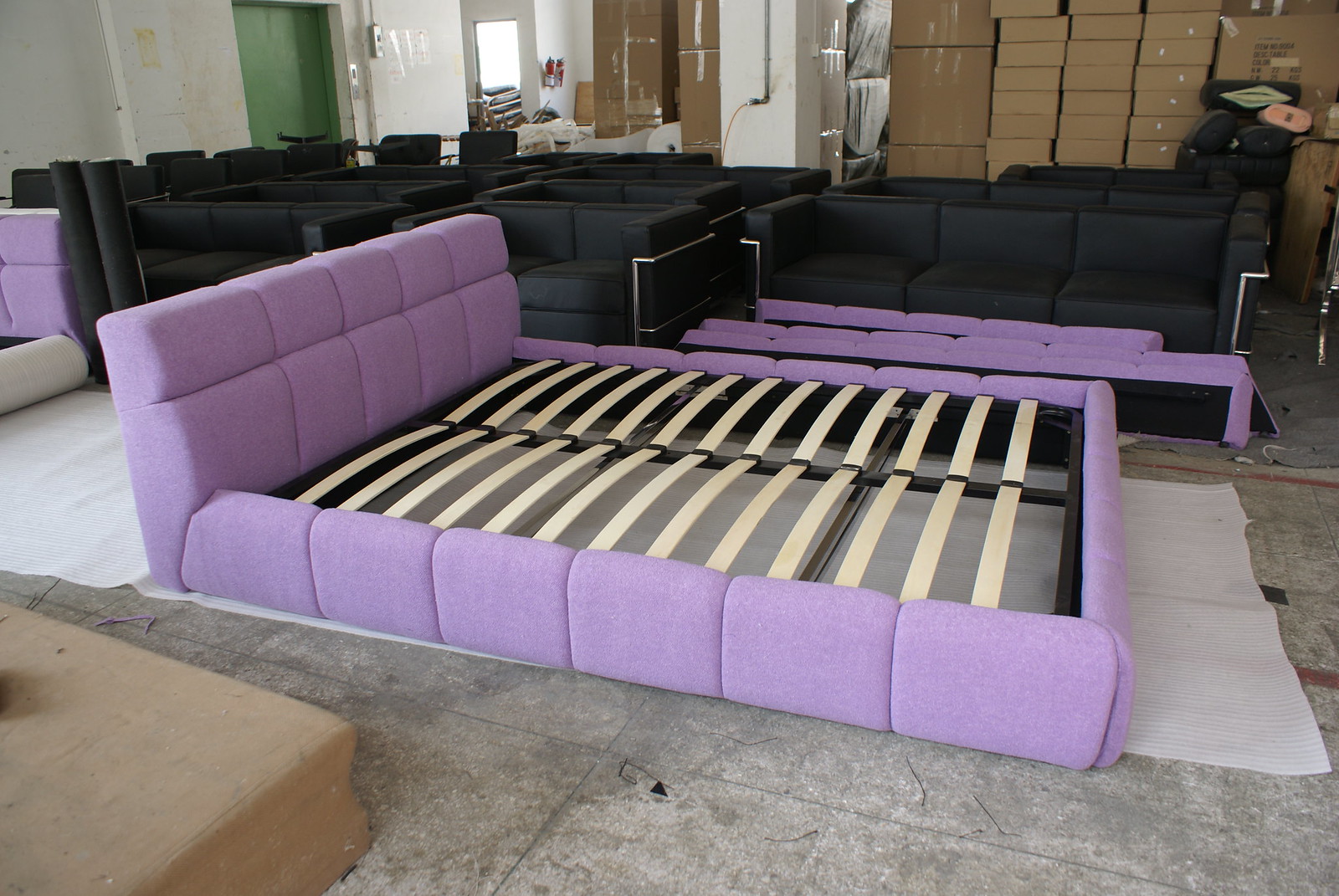The photo appears to be taken inside a furniture warehouse. In the foreground, there is a piece of furniture that looks like an extended couch, resembling a bed. This piece has a light lilac purple hue on the top and exterior, while the interior surface features black fabric accented with tan stripes. The item looks like it's still under construction, with its side panels distinctly purple. Surrounding this focal piece, there are additional purple elements, creating a color theme.

Positioned on what appears to be a stone floor with white sheets laid under them, the setting further includes multiple black, modern-day couches in the background, notable for their silver outlining along the armrests. To the upper right side of the image, there is a stack of brown boxes, indicative of a storage or assembly area. A green door and light switches are visible on the white walls towards the back of the warehouse. There is also an orange-tan object in the lower left corner that remains unidentified.

The image overall provides a detailed snapshot of a furniture warehouse with active assembly and storage areas, highlighting a purple, convertible couch-bed amidst a backdrop of modern furniture and various warehouse elements.